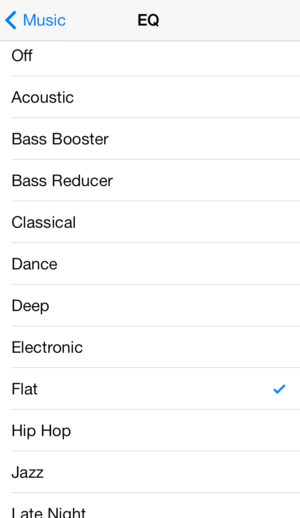The image captures a screenshot of an audio settings menu, likely from a music application or a smartphone. At the top left of the image, the word "Music" is displayed in bright blue text accompanied by a similarly colored arrow pointing left. Centrally positioned at the top, the letters "EQ" appear in black, all set against a gray background.

Beneath the "Music" label, a vertical list of audio preset options is shown, each separated by thin, light gray lines. From top to bottom, and excluding the "Off" option being at the start, these presets are arranged alphabetically: "Off," "Acoustic," "Bass Booster," "Bass Reducer," "Classical," "Dance," "Deep," "Electronic," "Flat" (which is marked with a blue checkmark indicating it is currently selected), "Hip Hop," "Jazz," and "Late Night."  The background of this section is primarily white, providing a clear contrast to the options listed. The space to the right of each word is left empty, likely to highlight the simplicity and clarity of the design. The area under the "EQ" label features subtle shading, adding depth to the visual layout. Overall, the interface is clean and organized, presenting an intuitive selection of sound profiles to enhance the listening experience.